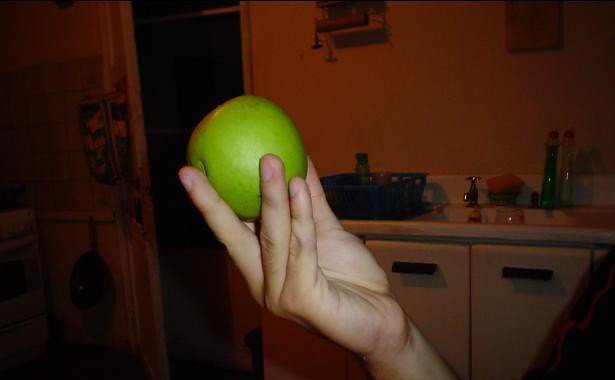In the image, the scene is set within a dimly lit kitchen, where a brown doorway with matching walls creates a cozy atmosphere. To the left of the doorway, a hanging skillet is affixed to a bar, hinting at its regular use. The door itself is adorned with a rack, from which various utensils are suspended. The other side of the doorway opens up to a view of the kitchen's work area: a light gray countertop equipped with silver faucets and knobs. Above the countertop is a spice rack, framing the space with an air of culinary readiness. Nearby hangs a framed picture in shades of brown, adding a touch of decoration.

On the countertop sits a small green bowl containing a red sponge, accentuating the kitchen's functional use. Prominently featured is a large blue basket, whose presence commands attention. Below, sleek cabinet doors reveal two handles. The focal point of the image is a hand emerging into the frame, holding a large, ripe green apple, its vibrant skin flawless except for the missing stem. The apple's bright hue contrasts with the darker, earthy tones of the surroundings, drawing the viewer's eye.